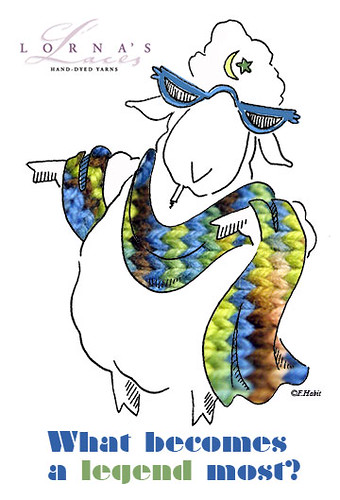The image depicts an anthropomorphic sheep standing upright, donning vibrant blue sunglasses perched on its forehead. The sheep is adorned with a detailed, multi-colored scarf—in shades of blue, green, and brown—draped across its body, cascading from its left arm, over its right shoulder, and looping around its right arm. A close-up, woven zigzag pattern is visible on the scarf. Atop the sheep's head rests a small turban decorated with a yellow crescent moon and a star. Below the sheep, in stylized blue and green letters, the caption reads, "What becomes a legend most?" The top of the image displays the phrase, "Lorna's Laces," in purple, alluding to Lorna's Hand Dyed Yarns.